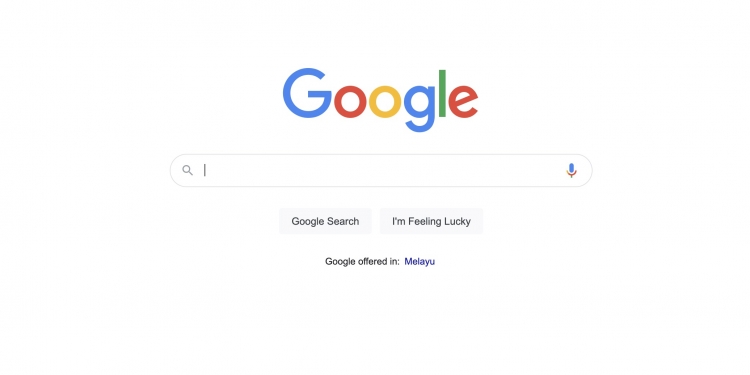The image shows a clean, minimalist layout of the Google homepage, typically seen when setting Google as the default search engine on a web browser. Dominating the center of the page is the iconic multicolored Google logo, spelled out with the letters 'G-O-O-G-L-E' in its recognizable blue, red, yellow, and green hues. Directly beneath the logo, there is a white search bar with a subtle gray outline. To the left of the search field, an illustration of a magnifying glass signifies the search function, while on the right, a microphone icon in Google colors invites users to conduct a voice search.

Below the search bar, two rectangular buttons in light gray hover just above the page's background, slightly standing out, yet blending subtly with the overall design. The first button is labeled "Google Search" and next to it, the second button reads "I'm Feeling Lucky" in black font.

At the bottom of the search box, a small note in blue text reads "Google offered in B-M-E-L-A-Y-U," suggesting the language setting is Malay. The rest of the page maintains a simple, white background, providing an uncluttered and user-friendly interface. The color scheme of the page includes white, black, various shades of blue, red, yellow, and green, with the link color differing slightly from the blue in the Google logo. The overall design is seamless, making it difficult to distinguish the white of the search page from the web browser's background, creating a cohesive look for the new tab interface.